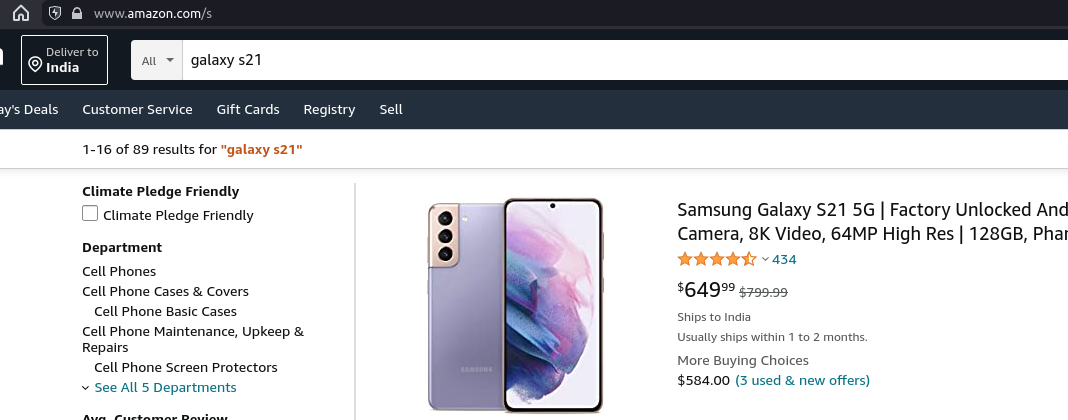Screenshot of an Amazon.com webpage displaying a search for "galaxy" in the search bar. The background features a sleek black and blue design. The top navigation bar includes links to Customer Service, Gift Cards, Registries, Sales, and Climate Pledge Friendly sections. Below these, various departments are listed: Cell Phones, Cell Phone Cases, Cell Phone Covers, Cell Phone Maintenance, and Cell Phone Screen Protectors. There's also a blue link that reads "See All 5 Departments." The main focus of the page is a Galaxy phone with an iridescent finish, prominently featured with three visible cameras. The phone is priced at $649.